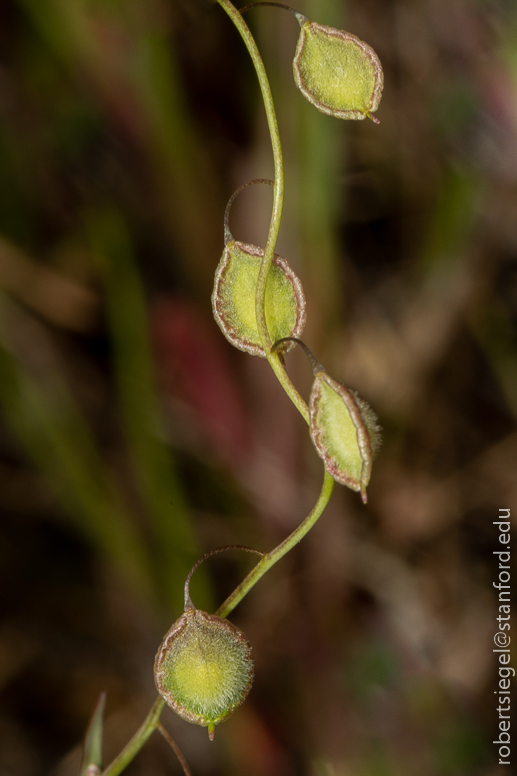This close-up photograph captures a thin, light green vine adorned with pod-like structures, curving gracefully from the bottom left corner, upward and to the right, before bending back to the left and exiting near the top center of the image. The vine showcases four distinct green pods, each characterized by an oval shape with a brownish-white outlining, adding a touch of contrast. The pod at the top features prominently, hanging downwards. Another pod is visible in the middle, with a short brown stem protruding from its top. A similar pod is located below and to the right of this central pod, seen from the side with a corresponding brown stem. The bottom left hosts yet another pod with a curling stem. The green vine itself is accented with subtle reddish-brown striping and tiny, fuzzy white flowers clustered around the pods. The blurred background hints at green and brown hues, possibly grass and soil, lending an outdoor, natural setting to the scene. A discreet white watermark at the bottom right, reading "Robert Siegel at stanford.edu," credits the photographer.